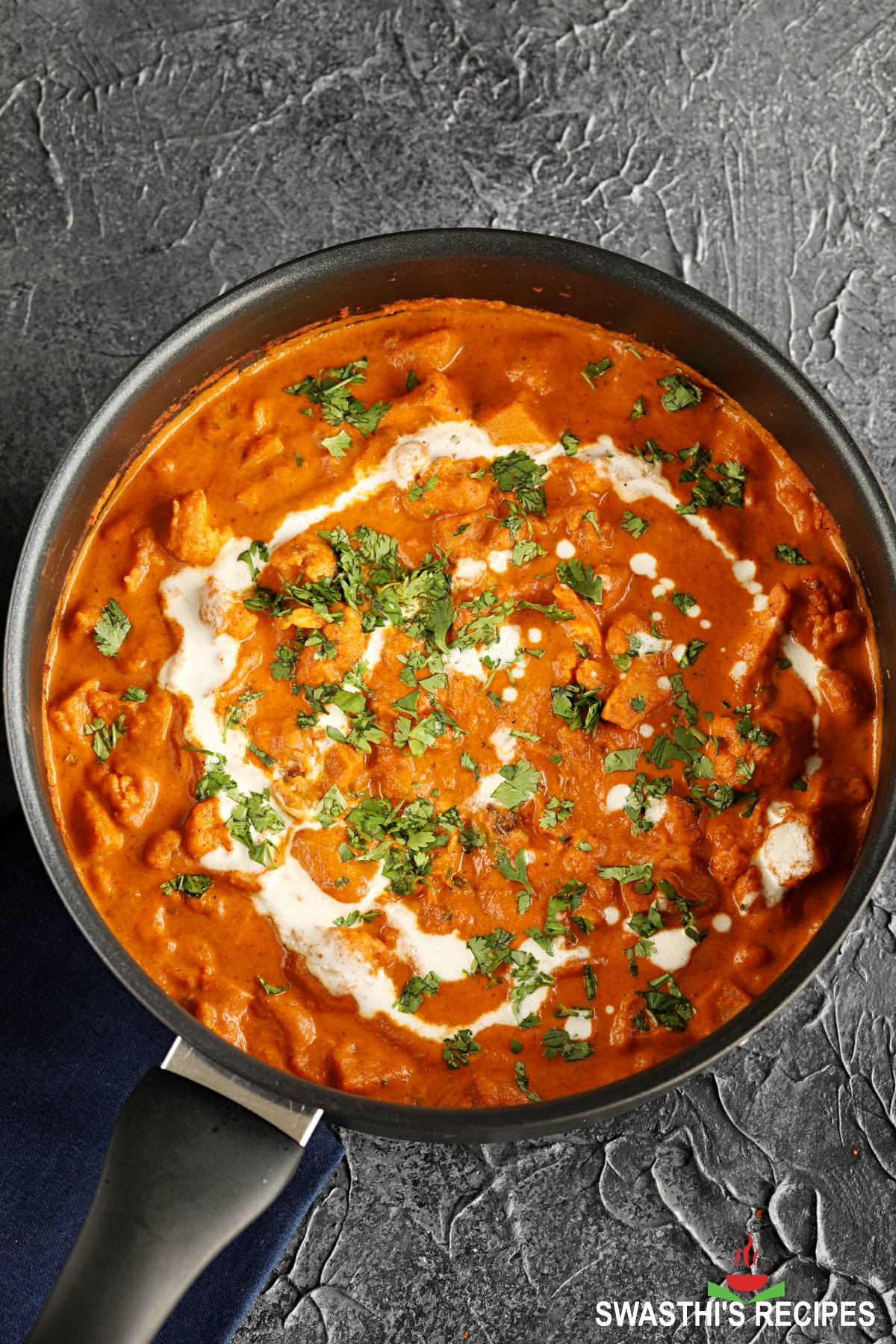The image is an overhead shot of a black metallic saucepan with a dark handle, placed on a gray tablecloth or a black and gray marble stone surface. The saucepan is filled with an inviting, tomato-based stew that is reddish-orange in color and contains chunks of meat, which could be either chicken or pork. The top of the stew is adorned with drizzled white cream creating a ring with droplets inside, and is garnished with bright green, crumbled fresh herbs, likely oregano or coriander. The overall look suggests it could be an Indian butter chicken or shakshuka. In the lower right-hand corner of the image, "Swathi's Recipes" is written in white font.